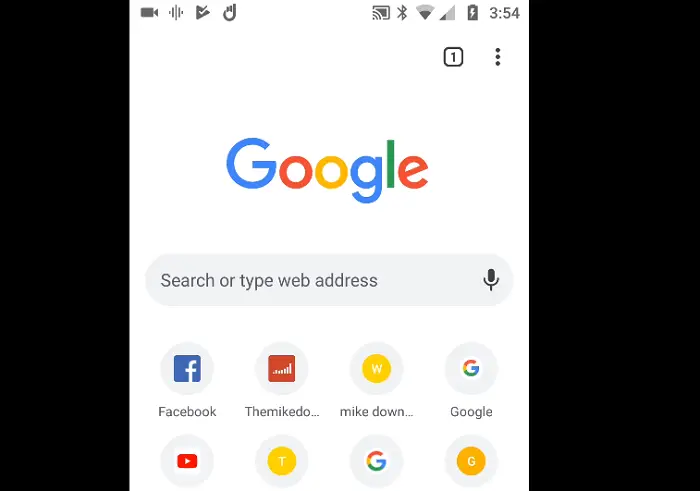The image features a Google homepage displayed on a digital device. The background is predominantly white. There are two vertical black bars on the screen, with the one on the right being wider. At the top right corner, the time reads 3:54. The battery icon indicates a decent charge, but the signal strength is relatively weak, though there is a web connection present.

On the left-hand side, four icons are visible. Centrally on the page, the Google logo is prominently displayed in its signature colors: blue, red, yellow, and green. Below the logo is the familiar search bar with the prompt "Search or type web address," accompanied by a gray microphone icon on the right side of the bar.

Below the search bar are several icons. The first icon is for Facebook, followed by another labeled Mic Do, and the next labeled Mic Down. There are subsequent icons for Google, YouTube, and one featuring a yellow circle with a "T" inside. Another Google icon follows, and the last icon is a yellow circle with a "G" inside.